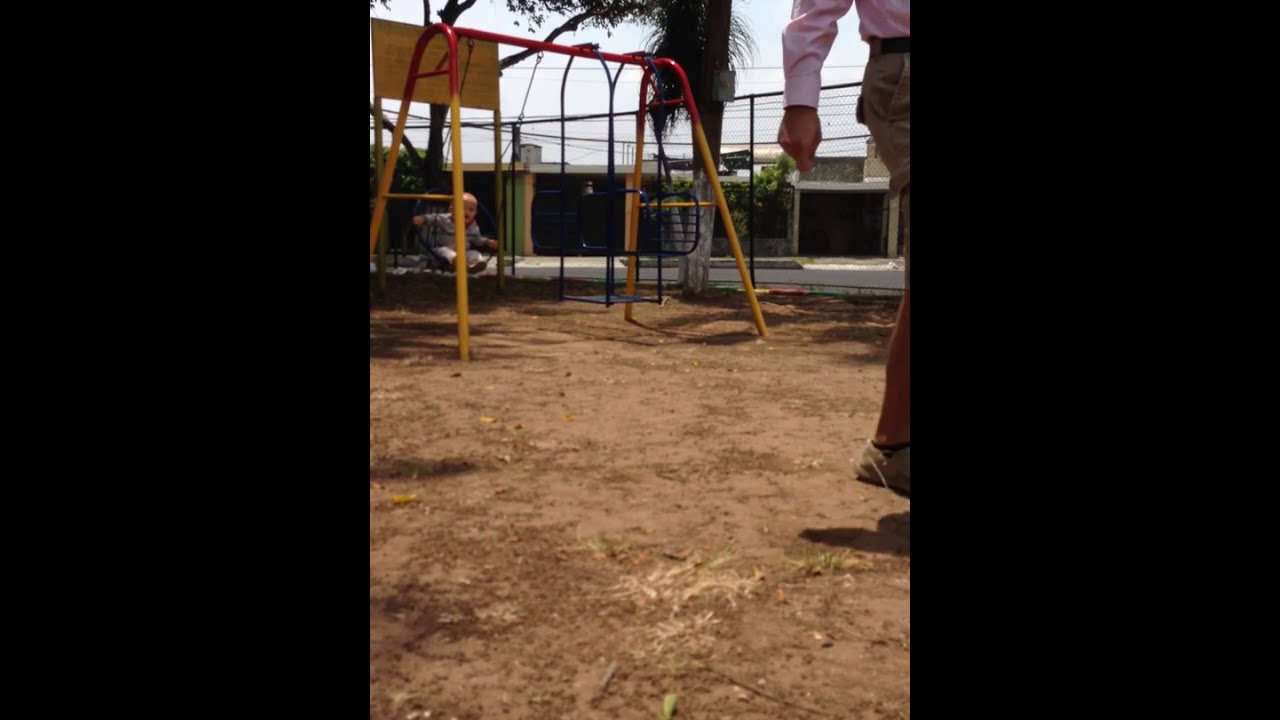The photograph captures an outdoor playground scene, dominated by a brightly colored swing set located in the upper left quadrant of the image. The swing set, which features yellow and red framework, includes two unique swings—a baby swing resembling a chair and a blue, accessible swing designed for individuals with disabilities. The baby swing is occupied by a baby, happily swinging.

The ground is primarily dirt, dotted with patches of dead grass, which adds texture to the scene. On the right side of the image, slightly above ground level, a person in business casual attire, including a white button-down shirt and khaki pants, is captured mid-jump, hovering about six inches off the ground. The individual’s attire is complemented by a belt and beige shoes, and their bare calf is visible.

In the background, a tall chain-link fence encloses the playground area, and beyond the fence, there are buildings that resemble a garage or car wash. The image provides a detailed snapshot of both the playground’s equipment and its surroundings, framed by a large black border on both sides.